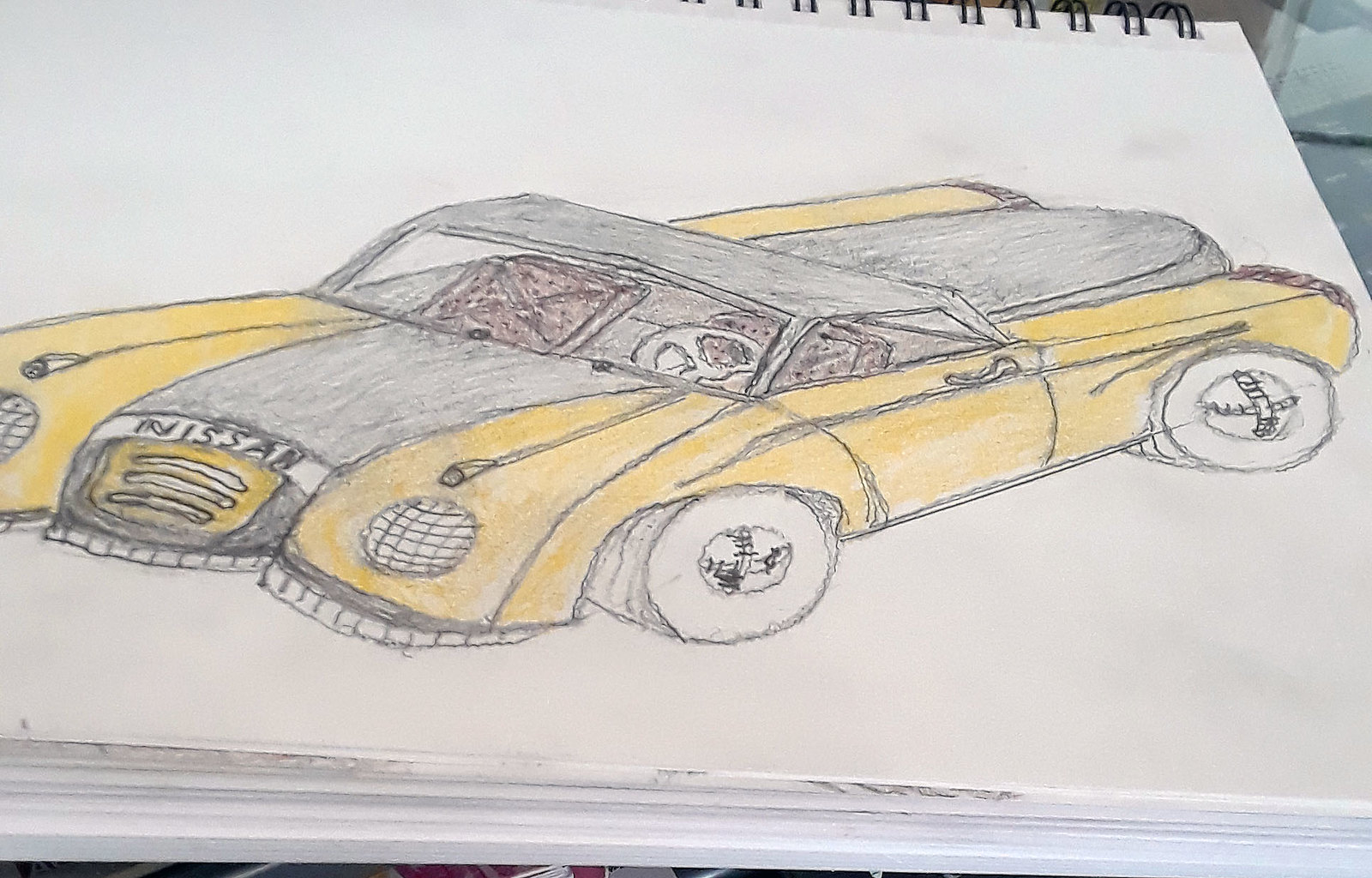A striking close-up photograph captures an artist's notebook from an extreme angle. The image is taken just at the cut edge of the notepad, with the spiral binding prominently displayed at the top, oriented in a slightly tilted landscape mode. The notebook rests on what appears to be the edge of a white shelf, providing a simple backdrop that brings focus to the artwork. Inside the notebook, a meticulous colored pencil drawing showcases a sleek, low-slung yellow vehicle, a single two-seater resembling a compact pickup truck. The front of this unique vehicle bears the brand name "Nissan," adding an authentic touch to the artist's rendition.